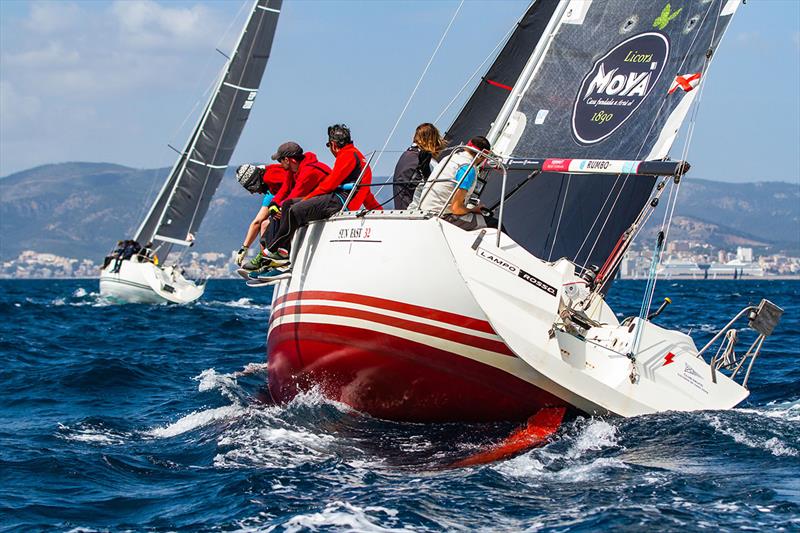This color photograph, taken outdoors during the daytime, captures two sailboats navigating choppy, deep blue waters against the backdrop of a beach city and mountain range under a hazy blue sky. The focal point is a white sailboat with black sails featuring the inscription "Lions Moa 1890." The boat, adorned with red pinstripes and a red keel, has at least six crew members on board. Two or three individuals sit with their legs hanging through the railing, wearing tennis shoes and red jackets. The crew members wear sunglasses and caps. The second sailboat in the background has a white hull and sails and also shows crew members engaging in sailing activities. The shoreline is lined with buildings, indicating an urban setting, and the mountains add a majestic layer to the scenic composition.